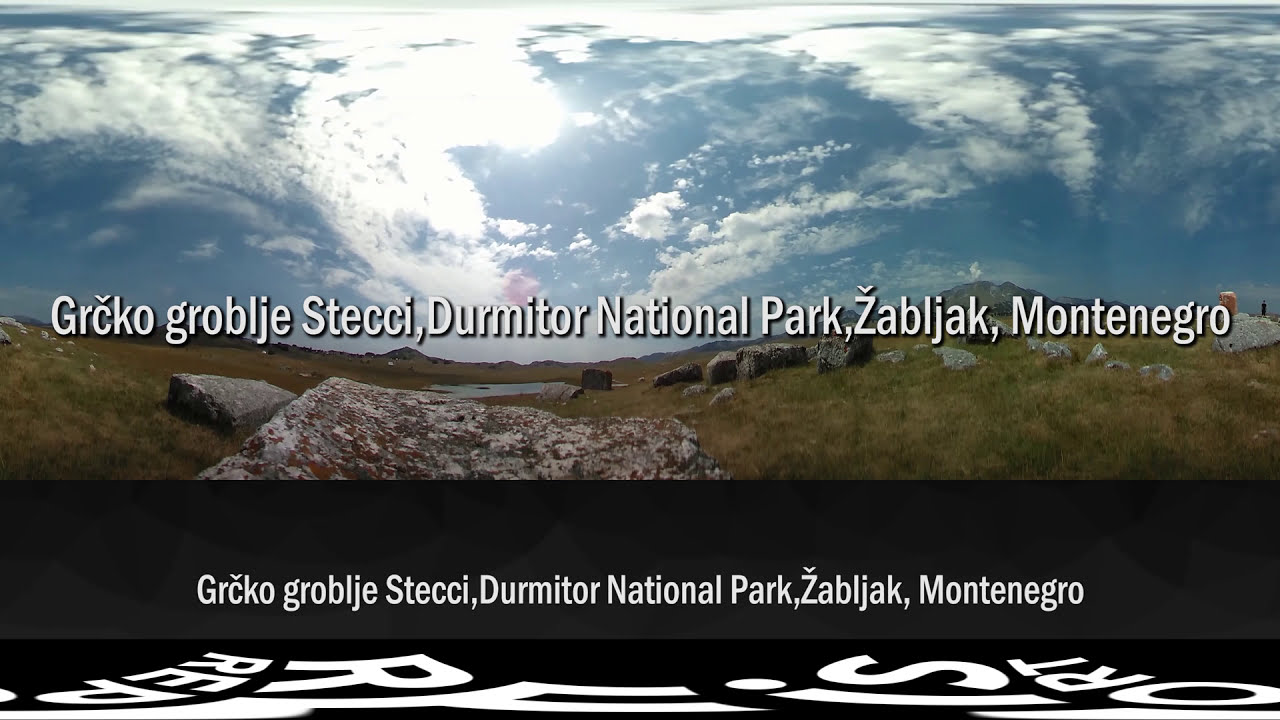The image is a detailed digital screenshot of an advertisement depicting Durmitor National Park, primarily focusing on a grassy hill landscape. At the bottom of the image, there are two banners with text, one in a foreign language and another including the word "Montenegro" clearly readable. A few lines of text also run across the center, although they are in an unreadable language. The landscape features a grassy field scattered with numerous rocks and stones, some appearing as large boulders or monolithic structures. A small pond or body of water is situated centrally within the scene. The sky occupies the top portion of the image, filled with clouds and suggesting an outdoor, midday setting. The colors in the image include shades of black, white, gray, tan, red, blue, and green, contributing to the natural and rugged atmosphere of the landscape.